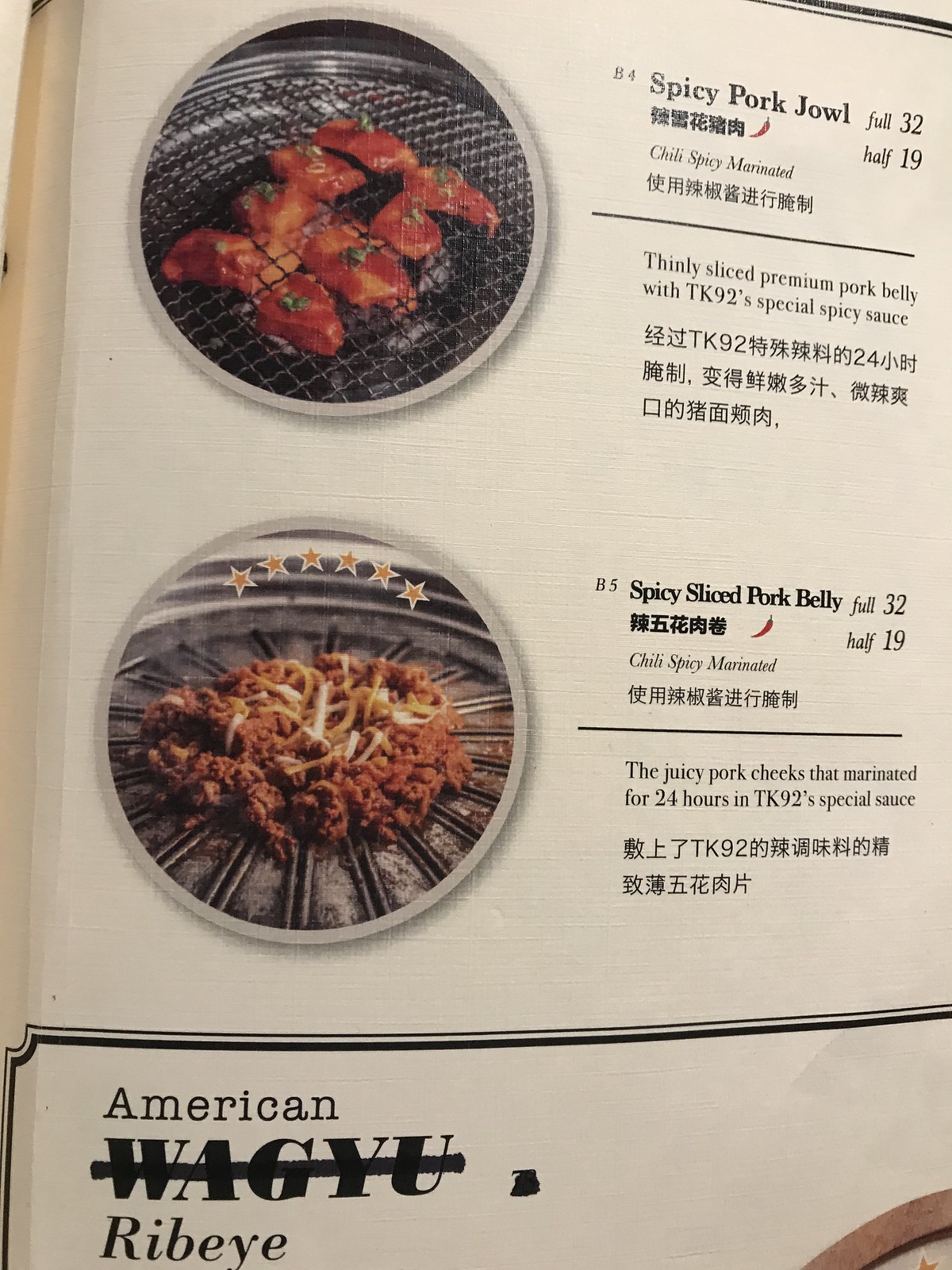This well-lit photograph captures a textured menu page primarily written in Japanese. The page features two circular photographs showcasing meal options. The top image displays eight pieces of meat sizzling on a grill. Adjacent to it, the detailed description reads: "Spicy Pork Jowl, Chili Spicy Marinated, Thinly Sliced Premium Pork Belly with TK-92's Special Spicy Sauce." Below, another circular photograph highlights very finely sliced or minced meat on a grill plate. The accompanying text states: "Spicy Sliced Pork Belly, Chili Spicy Marinated, the Juicy Pork Cheeks marinated for 24 hours in TK-92's Special Sauce." At the bottom, the text "American Ribeye" appears, with the word "Wagyu" crossed out by a marker.